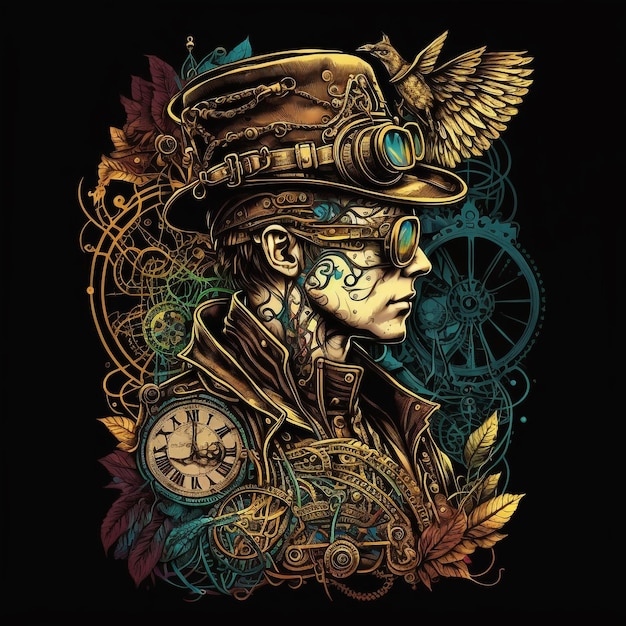The image presents a steampunk-themed illustration set against a black background. In the center, there is a detailed profile of a figure, who could be either a man or a woman, facing to the right. The figure wears a brown hat adorned with chains, buckles, and various metal fixtures, including a golden metal bird with a large tail seemingly perched atop or attached to the hat. The hat also features aviator goggles, despite the figure already wearing a second pair of goggles on their face. Their attire and accessories, such as wires and gears, contribute to a distinctly retro, industrial aesthetic.

Surrounding the figure, the background features various abstract elements like clock parts, mechanical dials, and brown leaves, all in shades of blue, green, yellow, and golden orange. A clock with randomized numbers adorns the lower left part of the image, contributing to the chaotic yet artistic composition. This amalgamation of steampunk elements and vivid colors gives the illustration an otherworldly, AI-generated feel, amplifying its unique, intricate design.